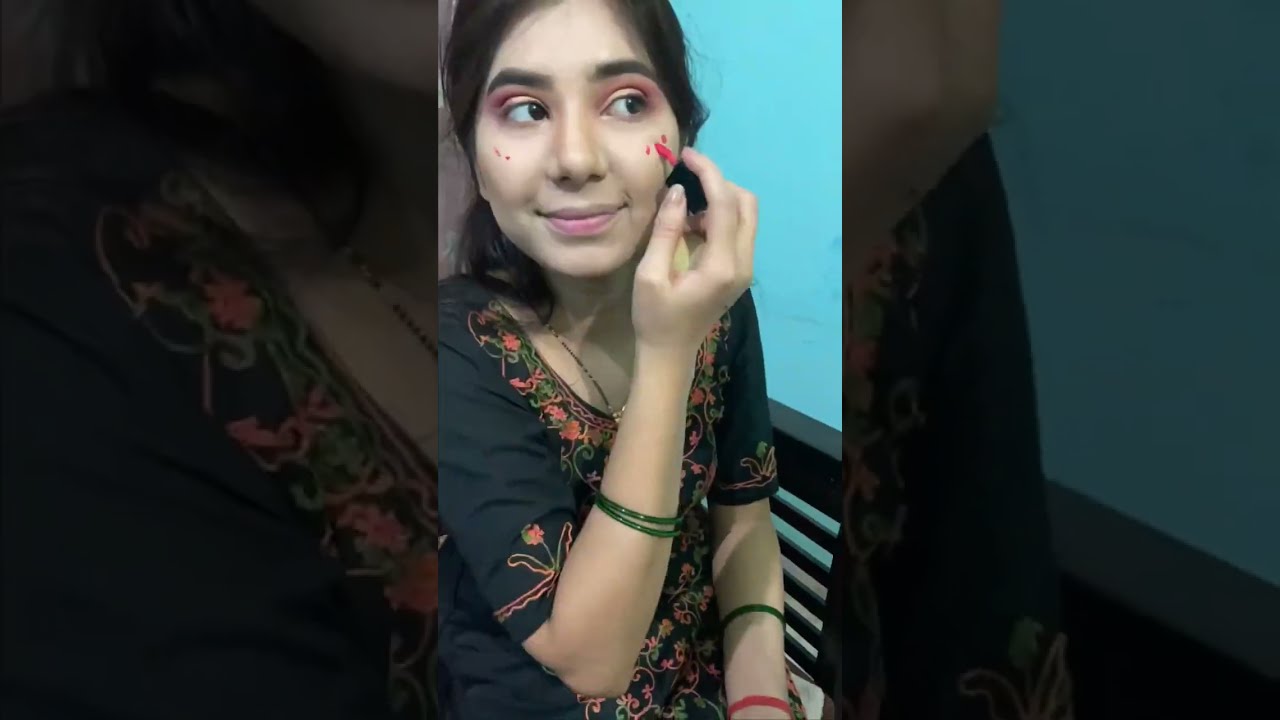The image displays a young woman, likely in her 20s and seemingly of Indian descent, captured in what appears to be a screen grab of a vertical video, possibly a makeup or fashion tutorial on TikTok. She has long, brown or black hair styled possibly in pigtails and is adorned in a black dress with ornate floral decorations around the collar, sleeves, and down the front. The background is a turquoise-blue wall or screen. Seated alone in a room, she is shown applying reddish-pinkish makeup dots to her left cheek with her right hand, while smiling gently and looking to the top left of the screen. Her eyes are accentuated with reddish eyeliner and she sports colorful armbands - one green and one red.